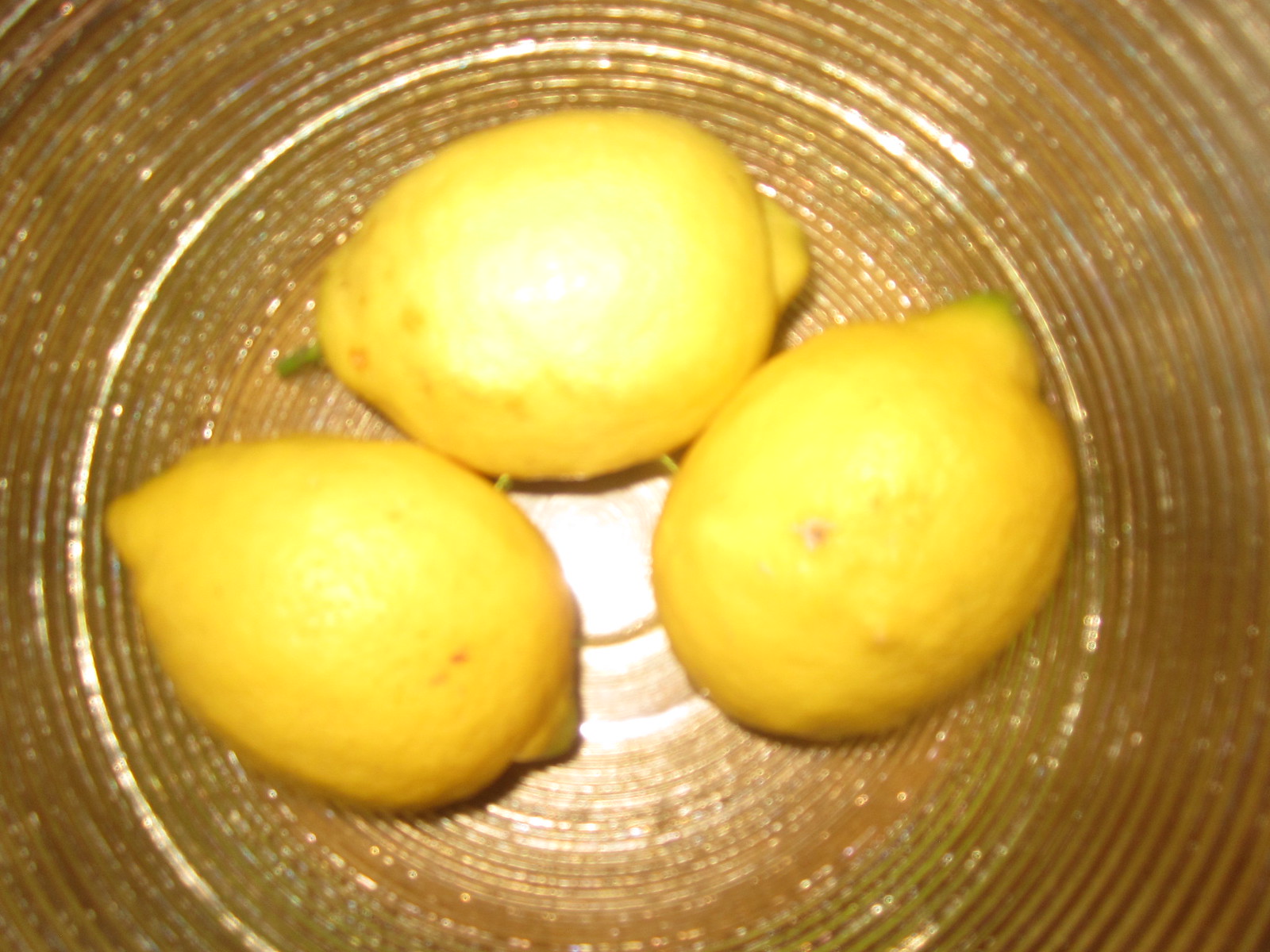This close-up photograph, taken with flash photography, depicts three unpeeled lemons arranged in a shiny, gold bowl with a spiral pattern composed of thin ridges. The image is blurry, likely due to the camera's unsuitability for close-up shots of small objects. The bowl's reflective surface creates significant white highlights amidst its intricate ridges. The three lemons are positioned with two at the bottom and one above them, forming a somewhat triangular arrangement. Notably, the bottom right lemon features a red spot, possibly a bruise, while the top lemon is vividly catching light, producing a prominent white splotch on its surface. Despite the blurriness, the lemons' yellow, bumpy texture is discernible.